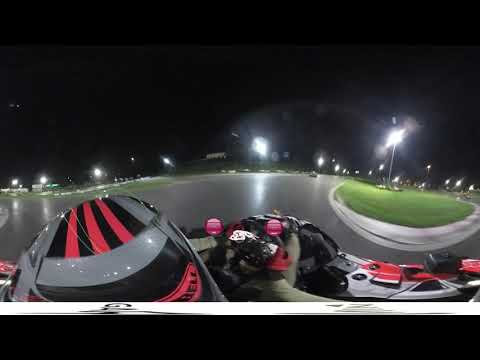The color photograph, captured at night, portrays a dynamic and somewhat blurry scene of a racetrack illuminated by numerous lights. The image, taken using a specialized panoramic filter with a fisheye lens, showcases a race car in motion, possibly a Formula 1 or Formula 3 vehicle. The scene is viewed from the cockpit, where the driver’s hands grip the steering wheel, and his legs are positioned on the pedals. The driver, wearing a helmet that appears gray-black with red stripe highlights, navigates the track. The car itself is predominantly red, white, and black, with hints of gray.

The racetrack, visible behind the car, is encircled by green grass islands bordered by white curbs and lines. A white strip with unreadable letters runs across the bottom of the photograph. Another race car, distant and indistinct in color, can be seen ahead on the track. The landscape orientation of the image accentuates the sweeping, nighttime vista, enhanced by the overhead illumination. The photograph’s blend of close-up and aerial perspectives gives it a unique, almost surreal quality, merging representationalism with the immersive effect of advanced photographic treatments.